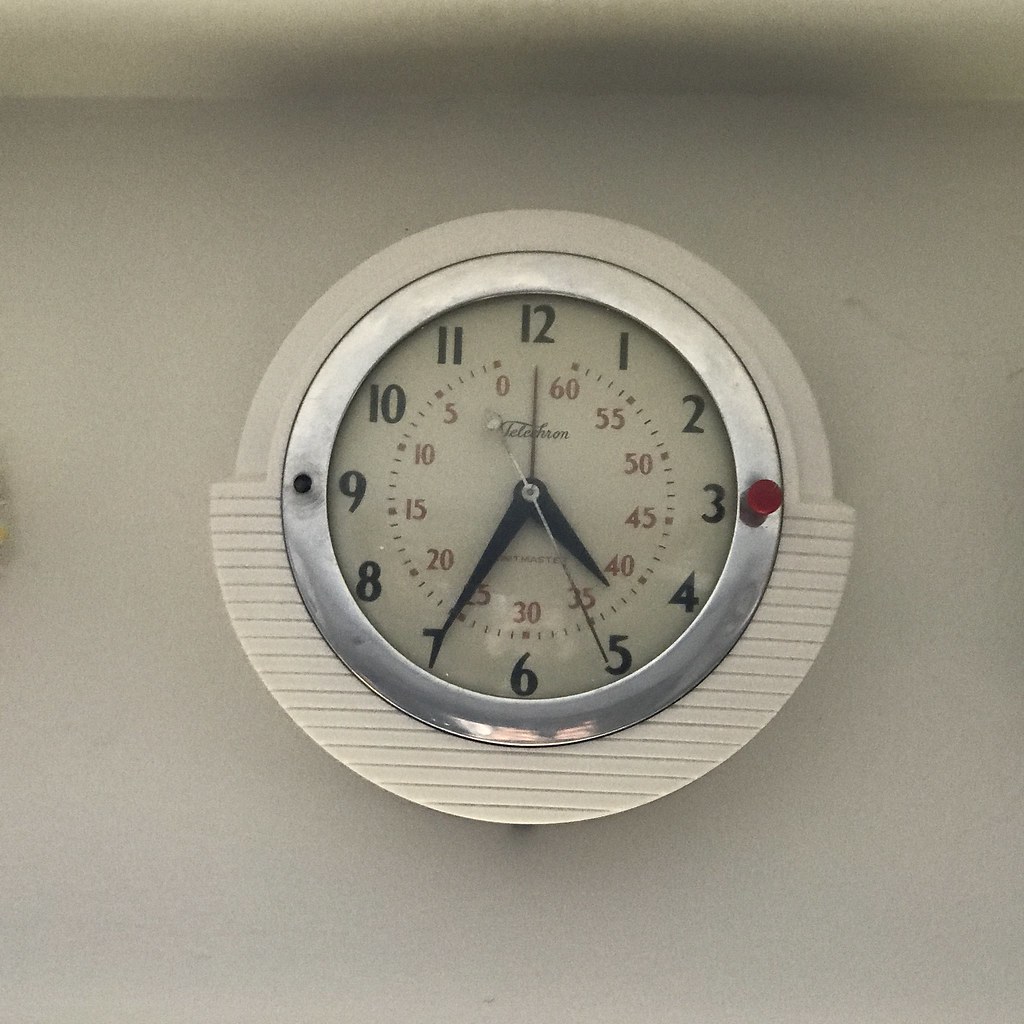In this detailed indoor photograph, we see a vintage analog clock, likely from the 1950s or 1960s, affixed to a plain white wall that has visible cracks, indicating its age. The clock features a circular design with a white plastic frame that becomes wider at the bottom, incorporating a stylized ribbed pattern. Inside this, a silver metal ring forms an additional interior frame. 

The clock face itself is white and features dual numbering systems: bold black numbers from 1 to 12 for the hours, and a secondary series of red numbers from 0 to 60 for the seconds, positioned on the interior of the clock face. Black minute markers are accompanied by red lines for the seconds. The hands of the clock are thick and black for the minute and hour indicators, with a silver second hand and a distinct brown hand for an alarm function. On the clock face, positioned at the 9 o'clock and 3 o'clock marks, there are small black and red dots respectively. 

The clock bears the logo "Telechron" written in stylized cursive. The room in which this clock hangs is dimly lit, creating an atmosphere that further accentuates the retro aesthetic of the clock.